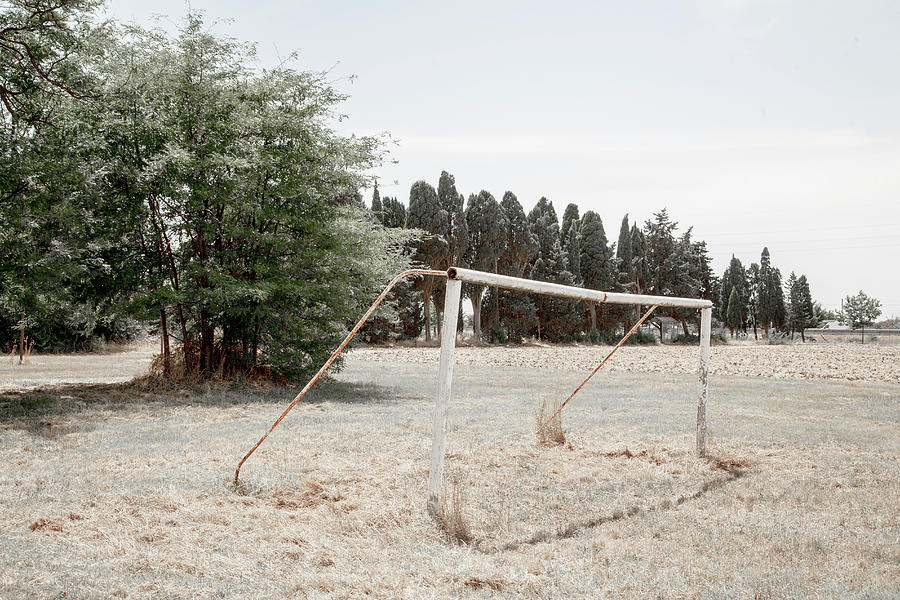The photograph captures a muted, vintage-looking scene of an abandoned soccer field under gray skies. The central focus is a derelict soccer goal post, which has lost its netting and now stands as a rusted metal frame. Originally painted white, the frame has deteriorated over time and is now covered in rust, especially prominent on the back parts and the two front poles. The frame is oriented with its opening facing the right side, while the back is turned to the left.

The field is overgrown with tall, unmanaged grass that has dried to a mix of muted green and tan shades. This unkempt grass covers the area around the poles, further emphasizing the sense of neglect. In the background, there is a row of trees, including both cone-shaped evergreens and a few standard-shaped trees, most notably positioned in the top left-hand corner. Some sections of the tree line stretch off into the distance, bordering what appears to be brown or dead agricultural land. This scene evokes a sense of abandonment and nostalgia, with the grey skies adding to the somber atmosphere of the deserted field.